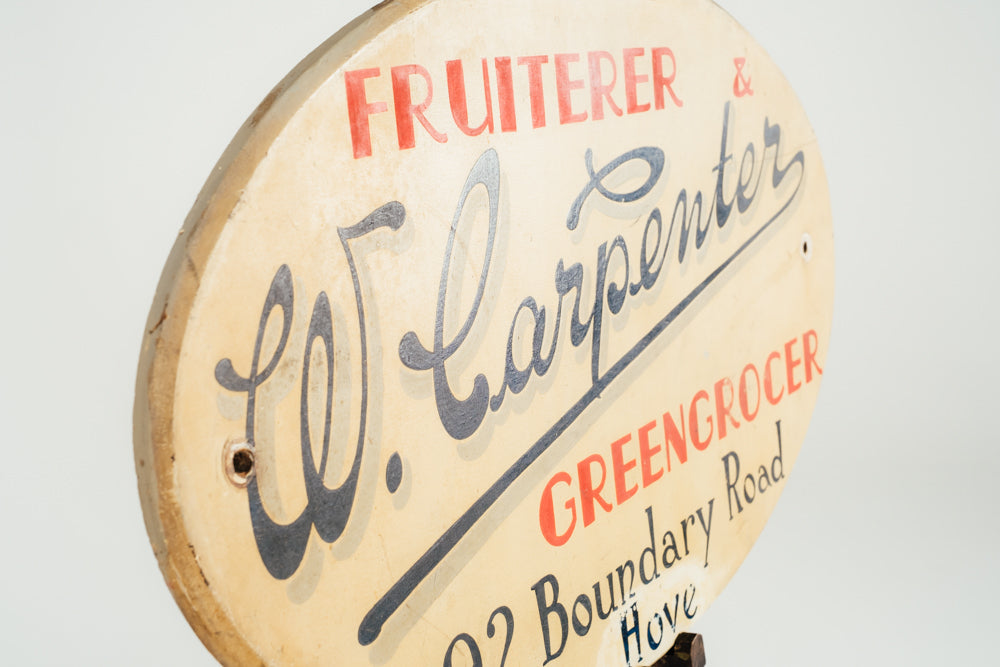The image features an angled, oval-shaped sign set against a white background. The sign is either metal or wood with a brownish-tan or cream-colored backdrop. At the top, in red lettering, it reads "Fruiterer." Below, in black cursive, it says "W. Carpenter," with the tail of the 'R' extending beneath the name. Further down, in red, it states "Green Grocer." The bottom part, also in red, provides an incomplete address: "Boundary Road, Hove." The sign has holes on the left and right edges for mounting purposes and displays an old-school aesthetic, using a mix of black and red fonts for the text. There is nothing else in the image.